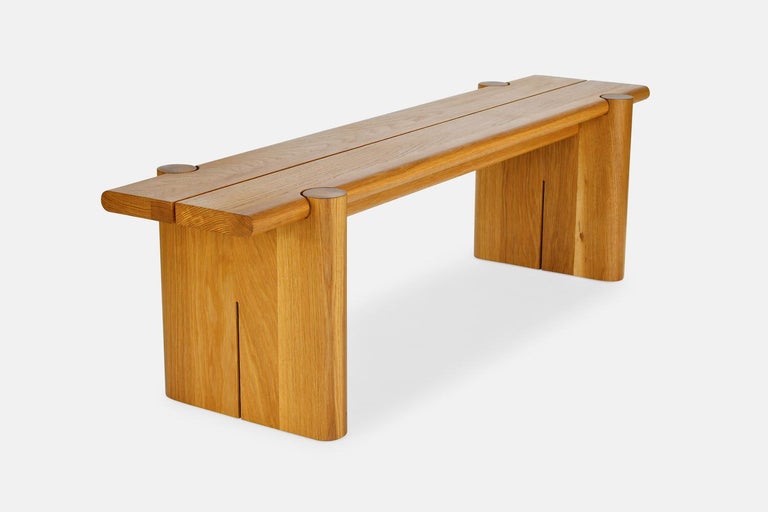The image features a sleek and modern Suleco bench by Last Ditch Design, positioned against a simple white-gray backdrop. The bench is crafted from light brown oak wood, exhibiting a polished, smooth, and glossy golden tan finish. The top comprises two long, rounded wooden planks joined together with a visible central line, showcasing the natural grain of the wood. The bench is supported by two sturdy wooden legs on either end, each shaped like broad, flat pieces of wood with round grooves at the top, curving inward to securely hold the seating planks. The design is minimalist, without any additional cushioning or decorative elements, emphasizing the elegant simplicity and craftsmanship of the wooden structure.